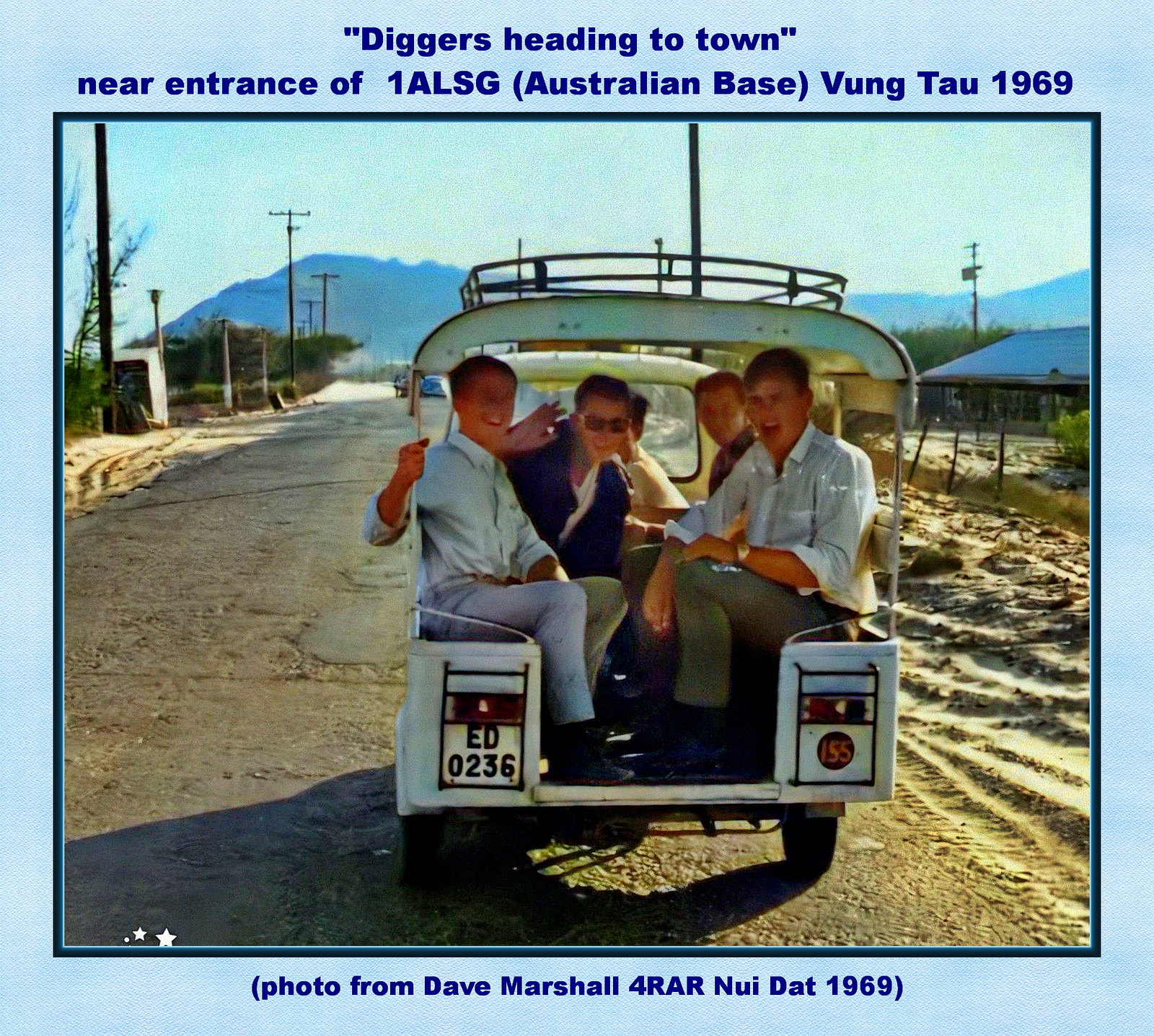This color photograph, framed with a light blue background and dark blue-lined borders, captures a nostalgic moment from 1969 at the entrance of the 1ALSG Australian base in Vung Tau. With text above the image reading, "Diggers heading to town," and a caption below noting, "Photo from Dave Marshall for RAR, Nui Dat 1969," the picture vividly showcases five men, likely soldiers, smiling and waving at the camera from the back of a rugged, open golf cart-type vehicle marked with the identifier ED0236. The road they are traveling on appears partially unpaved, with deep ruts and surrounded by sheds and telephone poles. In the background, the blue sky meets the silhouette of mountains, contributing to the scene's authentic and historic atmosphere.